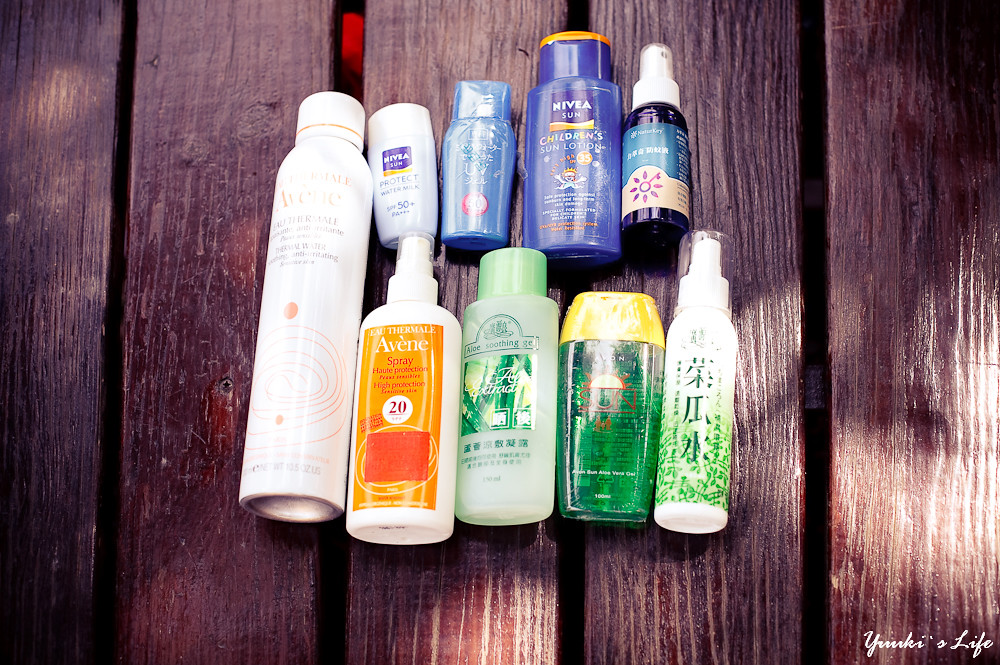The photograph showcases an array of sunscreen and sun protection products meticulously arranged on a rich, chocolate-brown wooden deck. The decking, characterized by thick planks and substantial gaps between them, appears to be varnished or stained. These gaps may serve a practical purpose, potentially allowing rainwater to drain through and prevent pooling on the surface, though it could also pose a risk of small objects falling through.

On the left of the image sits a tall, aerosol canister, likely a spray-on sunscreen or oil. Towards the top are two Nivea products: the Nivea Protect SPF 50 and the Nivea Sun Children's SPF 35, the latter adorned with an illustration of a child frolicking in the sun and surf. A smaller blue squeeze bottle is also visible nearby, alongside a dark brown, hard plastic bottle equipped with a spray top.

The bottom row features a variety of other sun protection items. There is a white spray bottle with an orange label from Avene, offering SPF 20 protection. Adjacent to it are three bottles with Asian writing. The central one, distinguishable by its yellow lid and see-through plastic containing a green liquid or gel, includes the word "sun" in its label. The two bottles flanking it are adorned with green hues and floral accents, with the rightmost bottle displaying Japanese characters.

This diverse collection of sun protection products suggests the individual might be reviewing them, possibly for their blog or website. This theory is supported by a white inscription at the bottom right of the image that reads "Yunkee's Life," indicating the content may be intended for Yunkee's blog, where she shares her insights and reviews on sun care products.